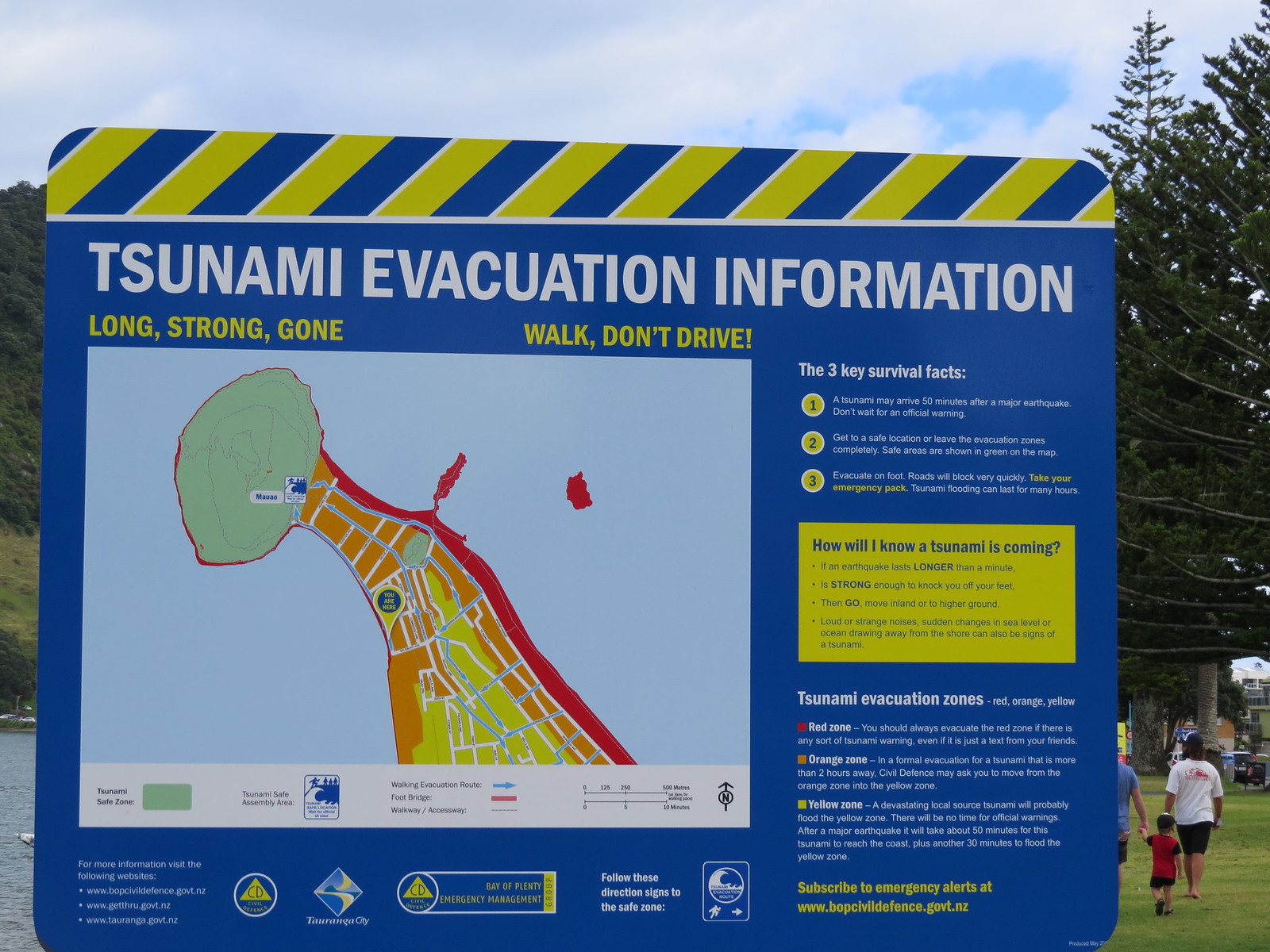The image depicts a large blue sign set in a scenic park area, indicated by the presence of grass, trees, and a water body with two adults and a child walking in the background. The top of the sign features a border with diagonal white, yellow, and blue stripes. Prominently displayed in white capital letters is the title "Tsunami Evacuation Information."

Beneath the title, two important instructions are highlighted in yellow text: "Long. Strong. Gone." and "Walk, Don't Drive." The left side of the sign contains a detailed map illustrating evacuation zones. The map uses a color-coded legend: red indicates areas most affected by a tsunami, orange shows moderately affected areas, and yellow represents the least affected zones. Green marks the tsunami safe zones. The map also includes markers for walking evacuation routes (blue arrows), footbridges (red lines), and walkways/access ways (black dotted lines).

On the right side of the sign, key survival facts are outlined:
1. A tsunami may arrive 50 minutes after a major earthquake. Don’t wait for an official warning.
2. Get to a safe location or leave the evacuation zones completely. Safe areas are shown in green on the map.
3. Evacuate on foot. Roads will block quickly. Take your emergency packs. Tsunami flooding can last for many hours.

A yellow box titled "How will I know a tsunami is coming?" lists indicators such as:
- An earthquake lasting longer than a minute or strong enough to knock you off your feet.
- Loud or strange noises and sudden changes in sea level or the ocean drawing away from the shore.

Additional information is provided about the tsunami evacuation zones:
- Red Zone: Always evacuate if there’s any tsunami warning.
- Orange Zone: Civil defense may ask you to move during a formal evacuation for tsunamis more than two hours away.
- Yellow Zone: Devastating local tsunamis will probably flood this area swiftly post-earthquake.

The sign concludes with website links for more information: www.bopcivildefense.govt.nz, www.getthrough.govt.nz, and www.tauranga.govt.nz, alongside logos promoting civil defense and the Bay of Plenty Emergency Management Group.